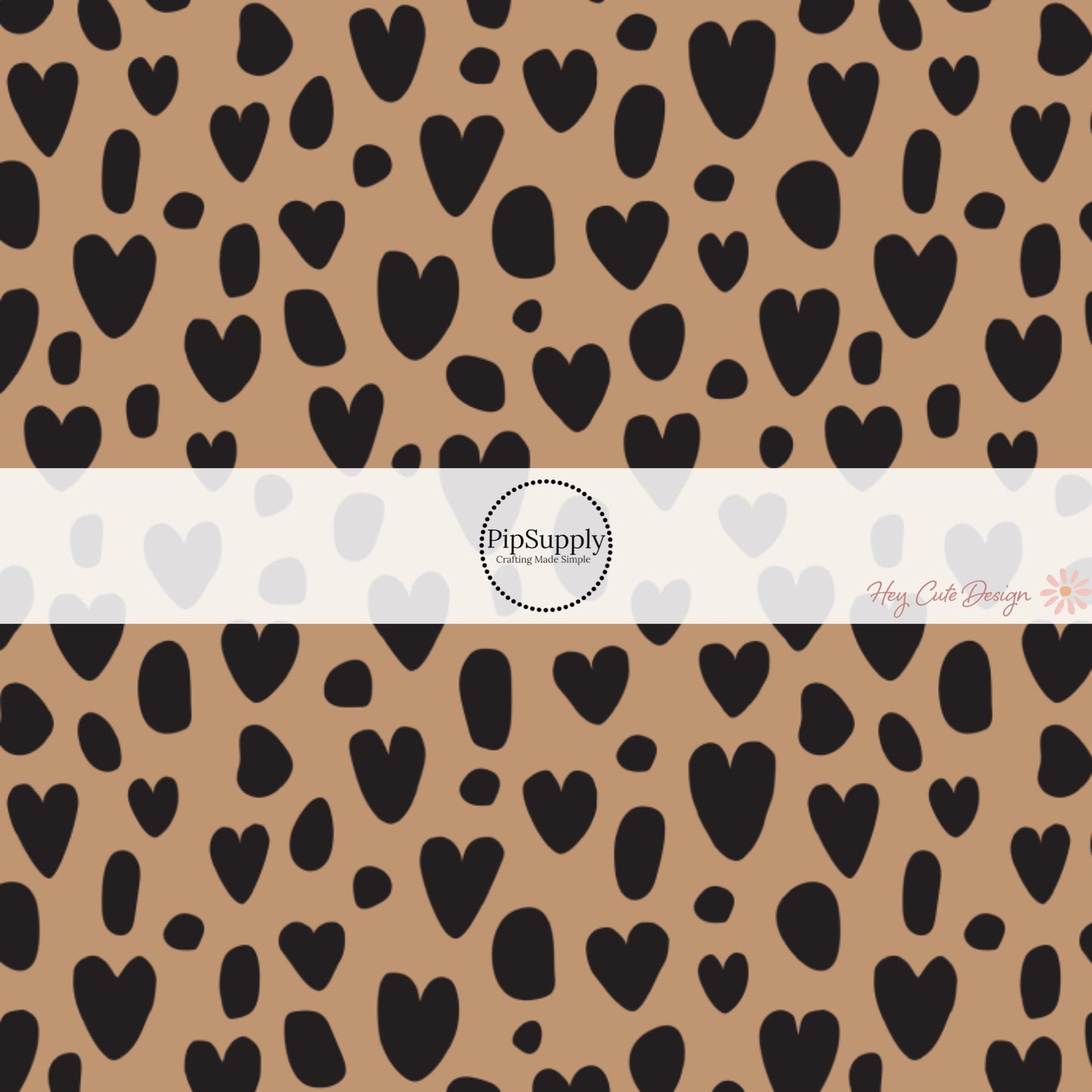This image showcases a piece of brown crafting paper adorned with an intriguing pattern of black hearts and dots, evoking a resemblance to cheetah skin through its unique arrangement and coloration. Central to the composition is a white horizontal stripe, intersecting the paper. Within this stripe sits a circular emblem bearing the text "PIP Supply, P-I-P-S-U-P-P-L-Y, Crafting Made Simple." At the bottom right of this banner, the phrase "Hey, cute design" is elegantly inscribed in pink script, complemented by a delicate illustration of a pink flower. The image is devoid of any human presence, focusing entirely on the design elements.